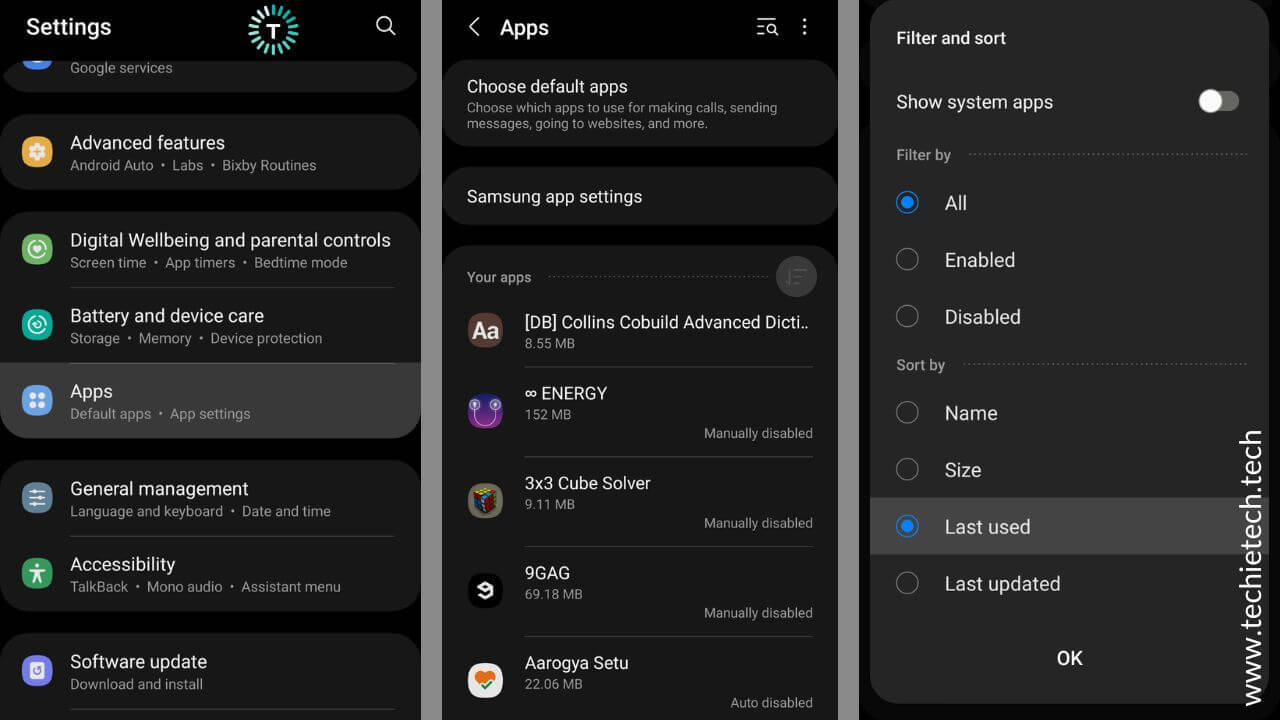The image displays a series of three screenshots taken on an Android smartphone running in dark mode, which features a black background. Here's an in-depth breakdown of each screenshot:

1. **First Screenshot:**
   - **Header:** The top section reads "Settings" on the upper left corner, next to a circular icon containing a "T".
   - **Search Bar:** Below the header, there is a search bar.
   - **Menu Options:** Several menu items are listed:
     - "Advanced features"
     - "Digital Well-being and Parental Controls"
     - "Battery and Device Care"
     - "Apps" (this item is highlighted in gray)
     - "General Management"
     - "Accessories"
     - "Software Update"
   - **Icons:** Each menu item is accompanied by a small gray box with various colors (blue, green, yellow).

2. **Second Screenshot:**
   - **Nav Header:** The top shows an arrow pointing left with the label "Apps," a search icon, and three vertical dots.
   - **Title and Instructions:** 
     - "Choose default apps" is prominently displayed in white text.
     - Followed by a description: "Choose which apps to use for making calls, sending messages, going to websites and more."
   - **Sections:**
     - "Samsung app settings"
     - "Your apps"
   - **App List:** Below the sections, several apps are listed:
     - "Cowan's Co-Build Advanced Energy"
     - "3x3 Cube Solver"
     - "9GAG"
     - "Ergon Setu"

3. **Third Screenshot:**
   - **Filter and Sort Options:**
     - "Filter and sort" is prominently displayed at the top.
     - Below it, there is a toggle for "Show system apps."
     - A filtering section includes options:
       - "All"
       - "Enabled"
       - "Disabled"
     - Each filter option is accompanied by a circle, with "All" highlighted in green or blue.
   - **Sorting Options:** Listed options include:
     - "Name"
     - "Size"
     - "Last used"
     - "Last updated" (with "Last used" highlighted)
   - **Footer:** Repeatedly shows the URL "www.techytech.tech."

These screenshots provide a comprehensive peek into the smartphone's settings interface, emphasizing the organization and customizable options available for managing apps and system settings.